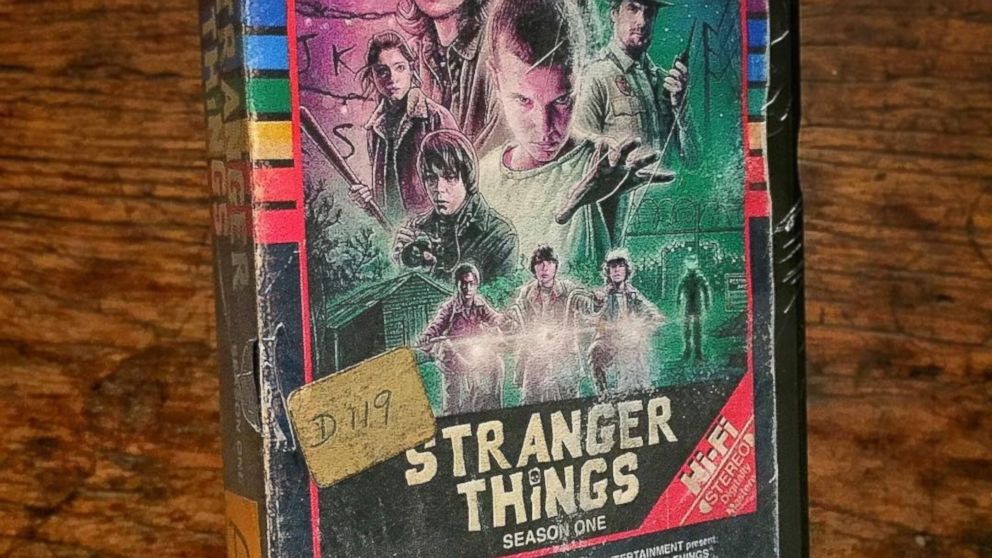The image portrays a vintage VHS tape of "Stranger Things" Season 1, set against an old, worn wooden table with noticeable divots and crease marks. The VHS tape, encased in torn plastic wrap, features vibrant cover art from the show's first season poster. Prominently, Eleven stands in the center with her buzzed hair and white shirt, extending her hand menacingly. Surrounding her are vibrant images of the rest of the cast, including a woman holding a bat and a man with a walkie-talkie. Below Eleven, three boys are seen riding their bikes with headlights on. The tape is decorated with rainbow-colored blocks along the top and right side, showcasing indigo, blue, green, yellow, orange, and red hues. An old sticker labeled "D119" and the text "Stranger Things Season 1 Hi-Fi Stereo Digitally Mastered" further emphasize its vintage charm.